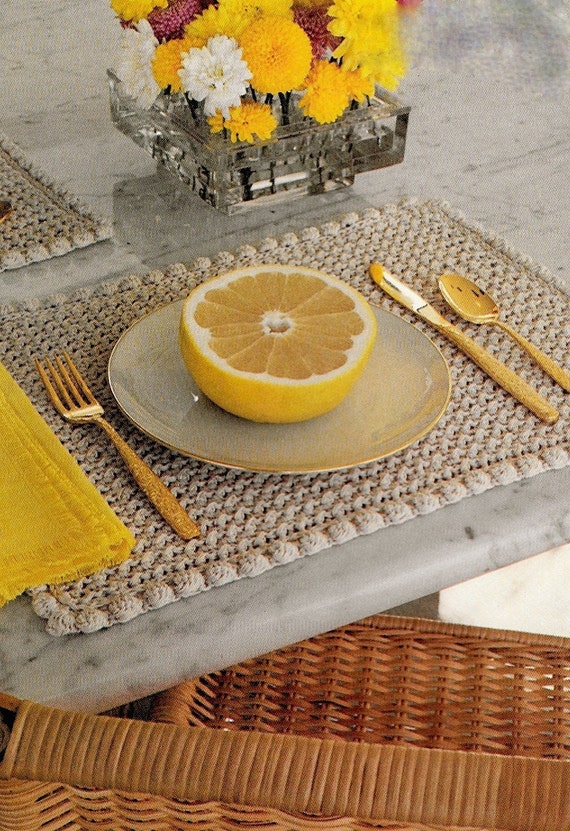The photograph captures a beautifully set breakfast table with a white and gray marble top. Central to the arrangement is a cut glass, flower arranging dish, displaying a vibrant mix of yellow, white, and red chrysanthemums. The table features knobby, crochet-looking placemats, with one prominently visible along the corner. On the left side of the setting, a mustard-colored cloth napkin rests next to golden-colored silverware, specifically a fork. Centered on a cream-colored plate is a halved yellow grapefruit, waiting to be eaten. The right side of the plate is flanked by a golden knife and spoon. Completing the scene is a cane-bottom wicker-style chair, pulled out and poised at the table's edge, adding a rustic touch to the elegant setting.